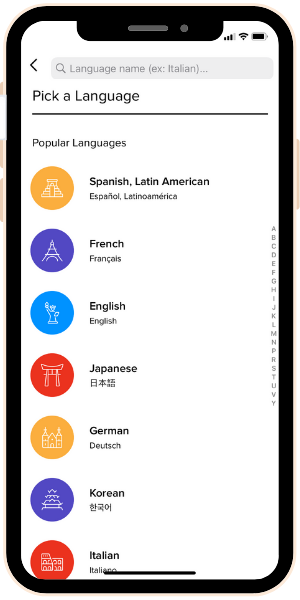This image features a detailed mock-up of a smartphone display, commonly used to demonstrate app interfaces or designs without the need for an actual device. The mock-up showcases a smartphone with a black bezel surrounding the screen. The top bezel features a notch with a grey oval denoting the camera and a small grey circle representing the speaker.

On the left side of the mock-up, there are buttons highlighted in a pink-orange hue. The screen itself displays a white background with various interface elements. At the top-right corner, icons denote the device's status: a cell phone signal showing three out of four bars, a full Wi-Fi signal, and a fully charged battery.

Just below these icons, a dark grey search bar is positioned, with a leftward-pointing black arrow beside it. The search bar features a magnifying glass icon and is labeled with "Language, name (e.g., Italian)...". Underneath this, in bold black text, the phrase "Pick a language" is displayed, followed by a bold black line.

Below this section, there is a list titled "Popular Languages." Each language is represented by a circular icon with a distinct silhouette and color theme:
1. **Spanish (Latin American):** Represented by a white temple-like icon within a circle. The text reads "Spanish, Latin American" in bold, with "Español, Latinoamérica" beneath it in regular black text.
2. **French:** Depicted with a white silhouette of the Eiffel Tower in a purple circle. The text reads "French" in bold, with "Français" underneath.
3. **English:** Illustrated with a white silhouette of the Statue of Liberty in a blue circle. Both "English" versions are simply labeled as "English."
4. **Japanese:** Shown with a white temple-like silhouette within a red circle, labeled "Japanese" with accompanying Japanese characters.
5. **German:** Represented with a white castle silhouette within a dark yellow circle, labeled "German" in bold, with "Deutsch" written underneath.
6. **Korean:** Featured with a white multi-tiered castle silhouette within a purple circle, labeled "Korean" with accompanying Korean characters.
7. **Italian:** Illustrated with a white villa silhouette within a green circle, labeled "Italian" in bold, with "Italiano" written underneath.

Overall, the mock-up offers a clear and organized view of how a language selection interface would appear on a smartphone.